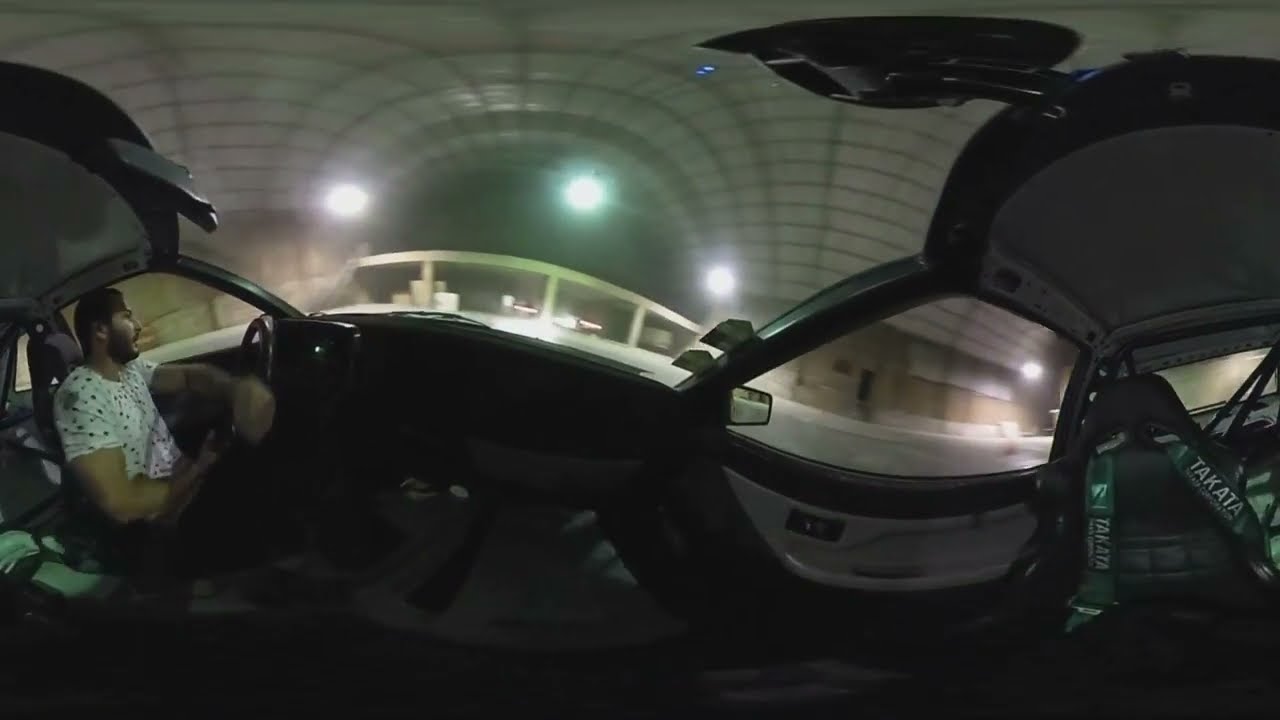Captured with a 360-degree panoramic fisheye lens, the image depicts an indoor scene, likely within a dimly lit parking garage or hangar at night. The environment is perceived as somewhat desolate and not inviting, characterized by a beat-up tan and lighter tan wall in the background, along with black and white ceiling rafters. A bridge or walkway with silver stairs and a gray or tannish top is also visible. The facility appears partially closed down, with just a few vehicles including a white truck and another indistinct car.

Inside the vehicle at the center of this scene sits a man looking to his left. He sports facial stubble, short-cropped hair, and a white t-shirt adorned with black polka dots or a motif. The interior of the car is mostly black with some gray accents, featuring racing bucket seats equipped with green seatbelts labeled TAKATA in white lettering. The floor mats are gray with the word MITSUI inscribed in black. Overhead lights illuminate parts of the structure and the car's see-through metal ceiling adds to the sparse yet industrial atmosphere.